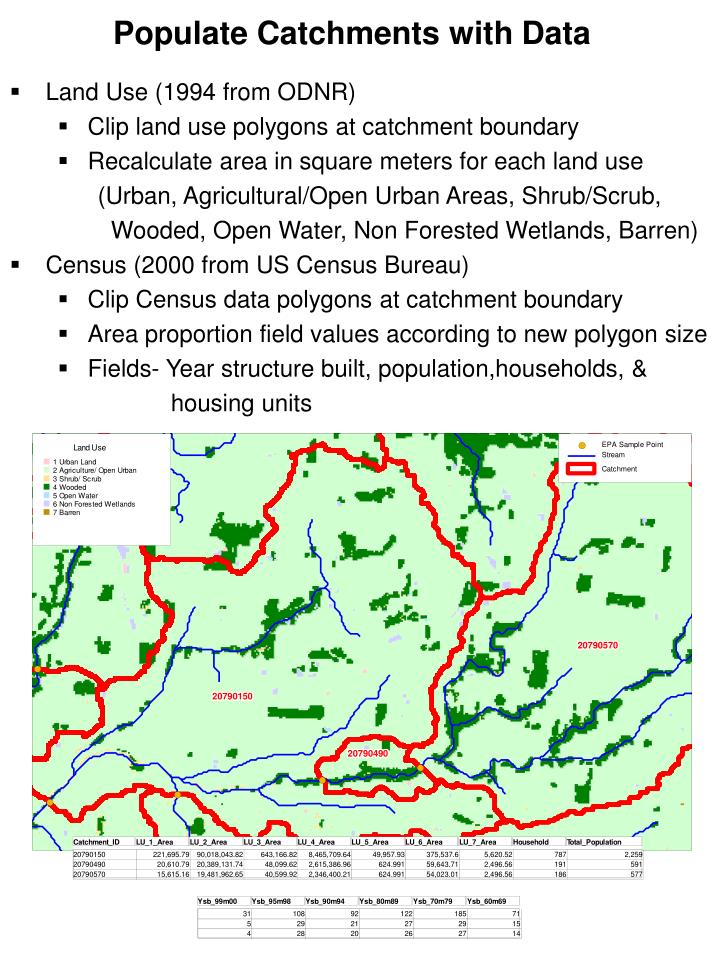This image features a detailed overlay of textual instructions above a comprehensive map. The text, set against a white background, provides a step-by-step guide for populating catchments with data from various sources. Key details include the specification of land use from 1994 provided by ODNR, with steps like clipping land use polygons at catchment boundaries and recalculating areas in square meters for different land use categories such as urban, agricultural, wooded, and barren areas. Similarly, census data from the 2000 US Census Bureau is processed by clipping census data polygons, adjusting areas proportionally based on new polygon sizes, and updating fields for year structure, population, households, and housing units. Below this text, the map visually represents the discussed data, featuring a green background interspersed with red lines marking catchments and blue lines indicating streams. The map also includes a legend that categorizes various land uses and details population statistics for specific areas, enriching the visual representation with essential geographic and demographic information.